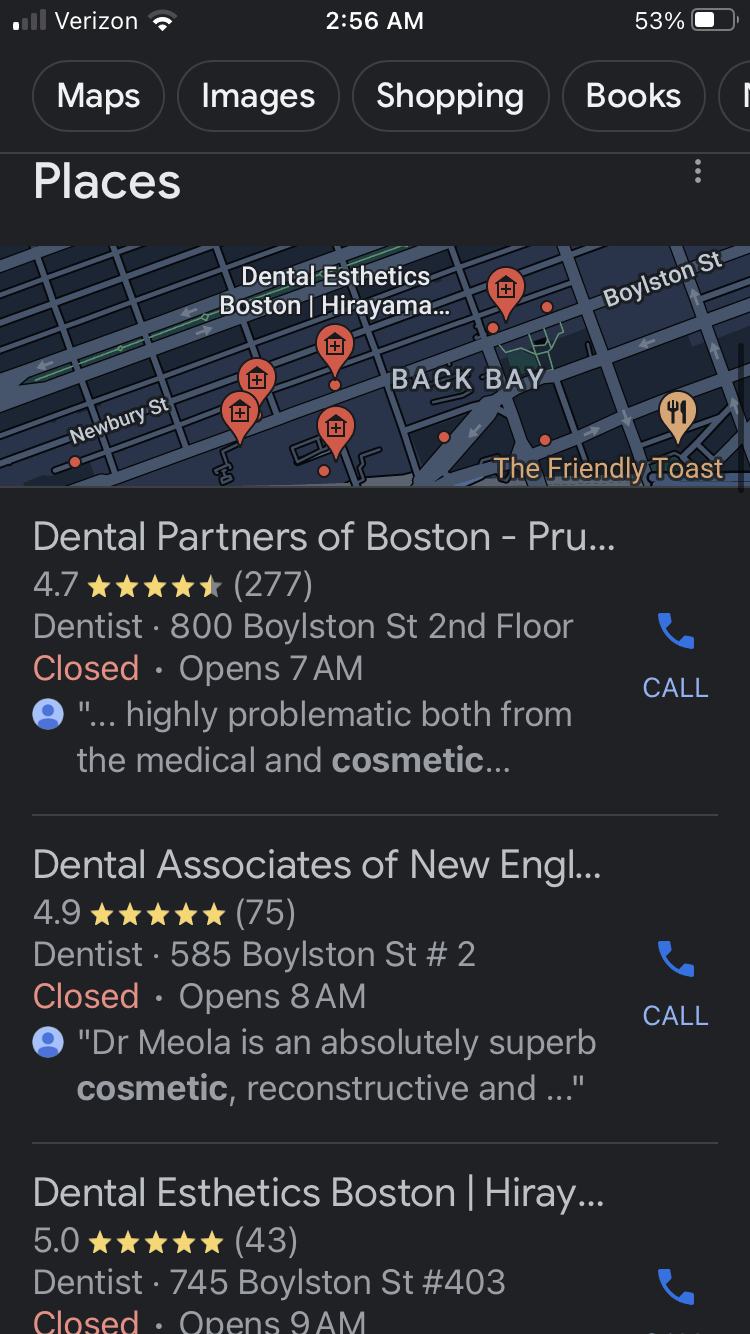The image, captured on an iPhone with a 53% battery at 2:56 AM, features several distinctive elements. The iPhone is powered by Verizon, boasting a full signal strength. At the top of the screen, there are navigation tabs in white reading "Maps," "Images," "Shopping," and "Books." Below these tabs, the word "Places" appears prominently. The main focus of the image is a map with a black background and gray streets, displaying various locations.

Highlighted on the map are several red pins marking the positions of "Boston Athletics" and "Dental Athletics Boston" offices. These locations are listed below the map alongside their specific street addresses: 745 Boylston Street, 585, and 800 Boylston on the second floor. Next to each listing, a blue phone handle icon with the text "Call" invites users to contact the offices. Additionally, patient feedback is noted under each office listing.

An orange pin and orange wording prominently highlight "The Friendly Toast," a nearby restaurant listed on the map. The image integrates essential details for each location, offering both contact information and patient feedback for user convenience.